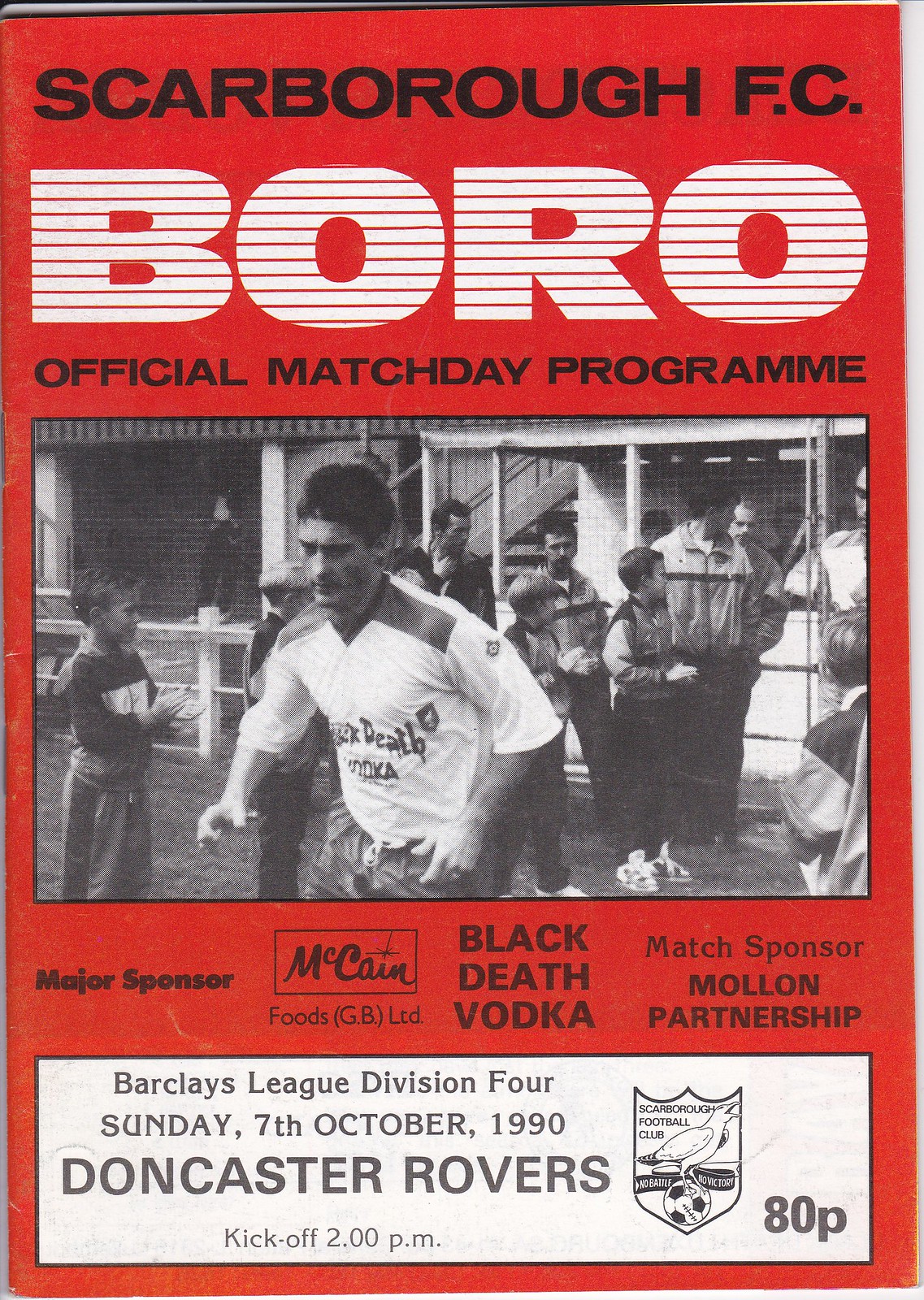The image is an advertisement for a Scarborough FC Borough Official Match Day Program, set against a red background. The top of the program features black text stating "Scarborough FC," followed by large white letters with red horizontal lines reading "Borough." Below this, in black text, it reads "Official Match Day Program," with the date Sunday, 7th of October, 1990, prominently displayed along with "Division 4," "Doncaster Rovers," and "kickoff 2 p.m."

Centrally, there is a black and white photograph taking up about half the program's height. It depicts a man in a white shirt, with his torso visible, moving towards the 7 o'clock position. His arms are bent at his sides, and he is looking down. Behind him are several children and men, appearing to be between the ages of 8-10 and adults respectively, possibly clapping and generally loitering. A white fence and what seems to be a concession stand or similar structure are in the background.

At the bottom of the program, various advertisements and sponsors are listed, including "McCain Foods," "Black Death Vodka," "Molen Partnership," and "GBLTD." The page reference is noted as Page 80.